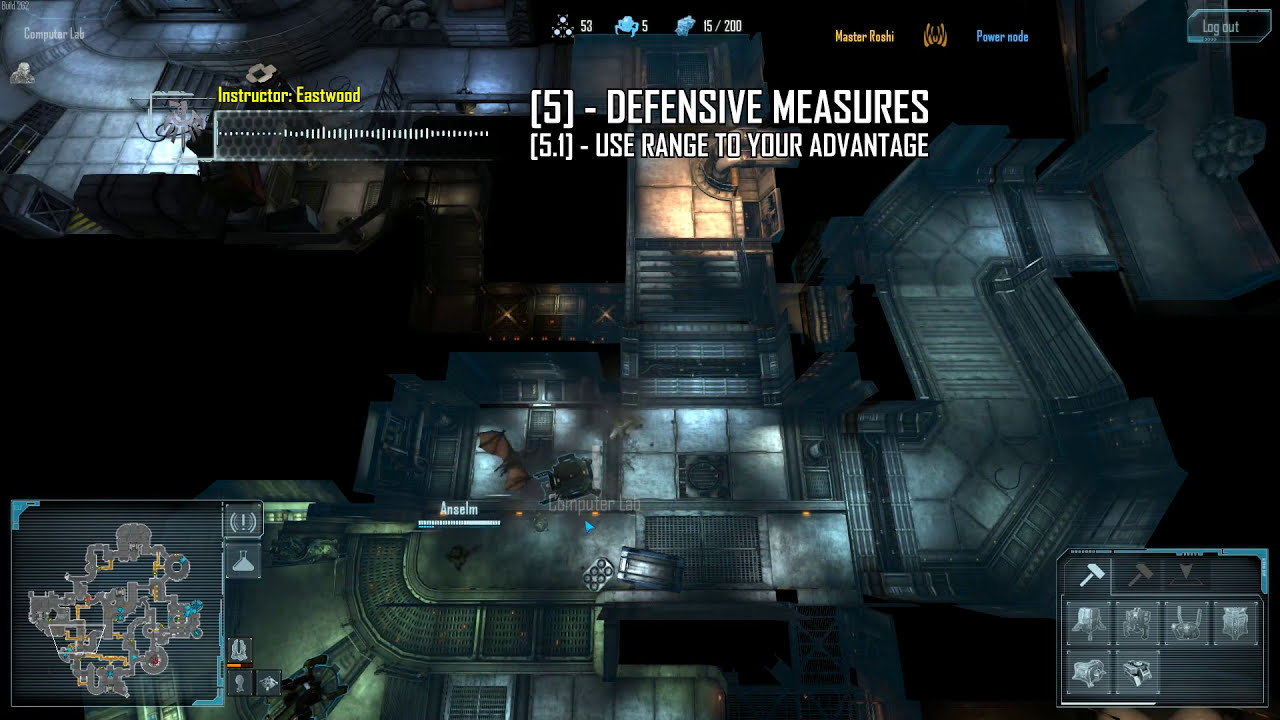The image depicts a screenshot from a strategy video game with a third-person, aerial view. The central character, named Anselm, navigates through a complex, industrial-style building that evokes the aesthetic of games like Metal Gear. The environment is dark and futuristic, with certain areas illuminated, revealing various paths and stairs. The top left corner displays the yellow text “Instructor Eastwood,” alongside a graph-like design. The upper center features game-related instructions in white text stating “Defensive Measures – Use Range to Your Advantage,” with the notations “5” and “5.1” accompanying the instructions. Additionally, a map of the area is situated in the lower left corner, while the bottom right corner features interactive elements or a key potentially indicating available weapons. The overall scene suggests a mission-focused gameplay scenario requiring strategic maneuvering and tactical decision-making.